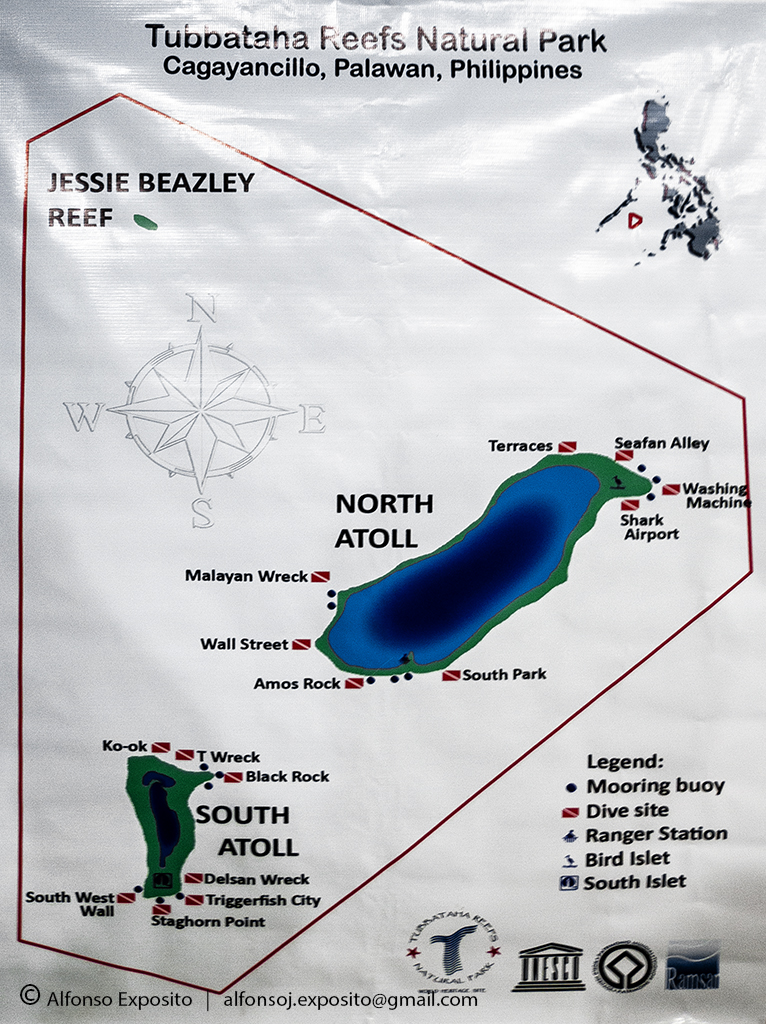This image depicts a detailed map of Tubbataha Reefs Natural Park in Cagayancillo, Palawan, Philippines, showcasing both North Atoll and South Atoll alongside several smaller areas. Key locations such as Jesse Beasley Reef, Terraces, Seafin Alley, Washing Machine, Shark Airport, Amos Rock, Wall Street, Malayan Wreck, K-O-K, T-Wreck, Black Rock, Delsan Wreck, Triggerfish City, Staghorn Point, and Southwest Wall are marked. The map features a directional compass for orientation and is color-coded with blue and green covering the two atolls, while black dots and red boxes denote landmarks indicated in the legend. The legend also details mooring buoys, dive sites, a ranger station, bird islets, and South Islet. The background is grey, and the map includes copyright information attributed to Alfonso Exposito, along with his contact email.